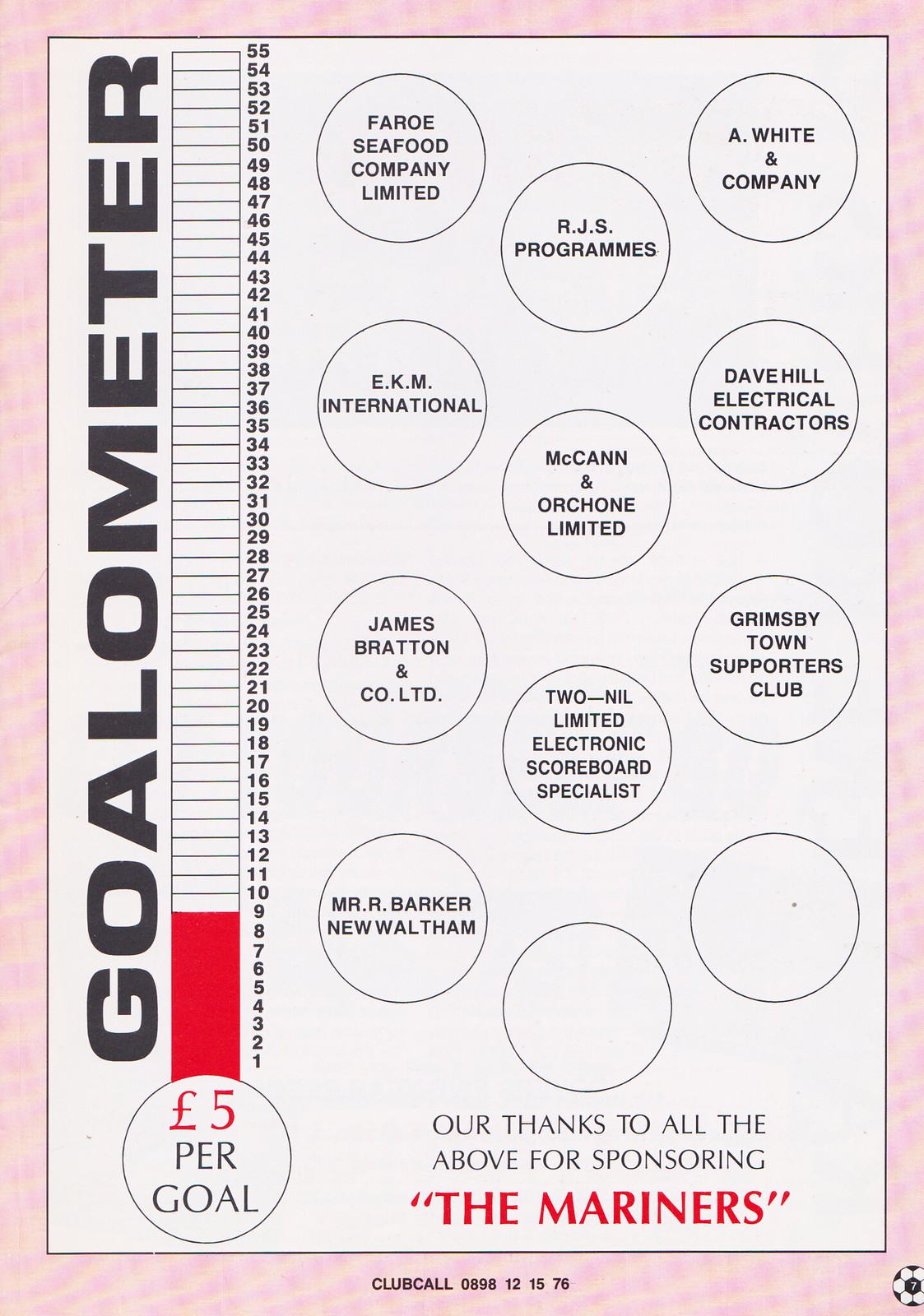This detailed portrait-oriented image features a soccer club program page with a light pink background, set within a yellow and black pinstriped border. Inset is a white rectangle. Along the left-hand side, vertically written in bold black type, is the word "GOAL-O-METER," all in capital letters. Adjacent to this, there is a thermometer-style meter marked from 1 to 55, displaying a red fill up to the number 9. Beneath this meter, a circle contains the text "5 Pounds per Goal" with "5 Pounds" in red lettering and "per Goal" in black.

To the right of the meter are 12 circles, each containing the names of sponsors in black type on a white background. Ten circles are filled with the names: Faroe Seafood Company Limited, RJS Programs, A. White & Company, EKM International, McCann & Orkin Limited, Dave Hill Electrical Contractors, James Bratton & Co. Limited, 2-NIL Limited Electronic Scoreboard Specialists, Grimsby Town Supporters Club, and MRR Barker, New Waltham. Two circles remain blank.

Below these sponsor names, a black text reads, "Our thanks to all the above for sponsoring" with "The Mariners" in red type and enclosed in quotation marks. The footer of the image, set against the pink and yellow background, includes a club contact detail "Club Call 0898-12-1576" and features a small black-and-white soccer ball emblem in the lower right-hand corner. The page is styled in a publication print format.